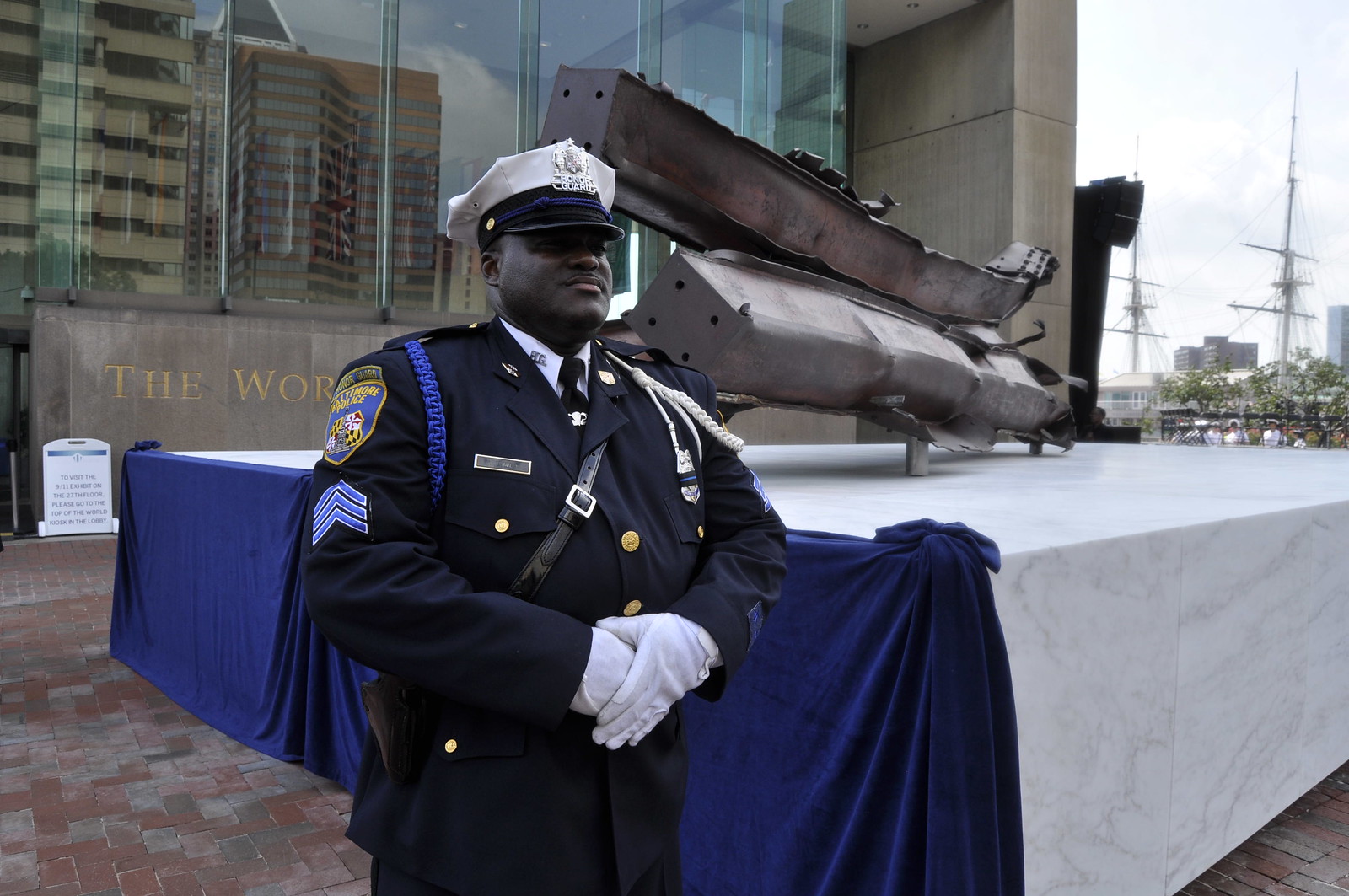The photograph captures an African American police sergeant in a full formal dress uniform, standing outside in front of a monument. The sergeant wears a dark blue uniform adorned with white gloves, a white shirt and hat, and a dark tie. His uniform features three blue stripes on the right shoulder, indicating his sergeant rank, and he has a leather strap across his chest. Additional adornments include a metal badge, name tag, and several pins, highlighting his distinguished status.

Behind the sergeant is a large stage with a white and blue cover, showcasing two substantial, damaged steel beams, likely remnants from the September 11th attacks. The beams, each approximately eight or nine feet long, are positioned one atop the other on the stage. A blue blanket drapes over the left side of the monument, suggesting it might be part of an unveiling ceremony. The setting includes a white cloth-covered area with white stone or brick at the base.

In the background, the building facade displays the partial text "WOR" beneath reflective windows that mirror tall buildings across the street. Further in the distance to the upper right, the masts of historic sailing ships pierce the sky, adding a maritime touch to the urban landscape. The scene reflects solemn remembrance and official honor.